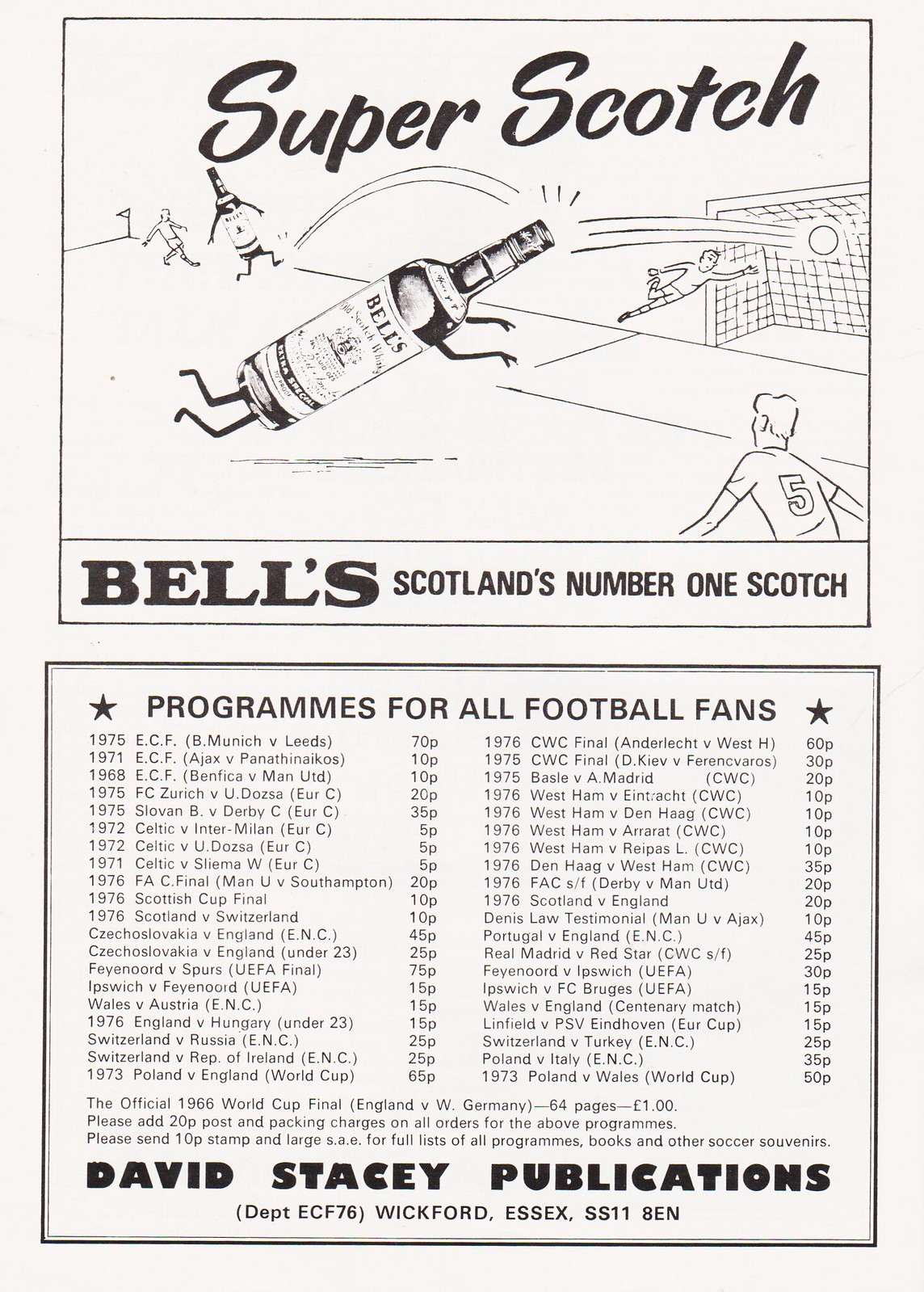The black and white image features two distinct advertisements. Dominating the upper half is a cartoon-style sketch promoting Bell's Scotch whiskey. The artwork depicts animated scotch bottles playing soccer, with one bottle kicking a ball that bounces off another bottle and into a net. The scene is accompanied by the slogan "Super Scotch" and the tagline "Bell's Scotland's number one scotch" in bold lettering. Below this, the advertisement transitions to a promotion for David Stacey Publications, targeting football enthusiasts. This section, tagged with the line "Programs for all football fans," outlines two lists: one for match programs and another for individual team programs, with the number of pages for each program listed on the right. The detailed organization suggests a variety of publications tailored to different games and teams, underlining the resourcefulness of David Stacey Publications.